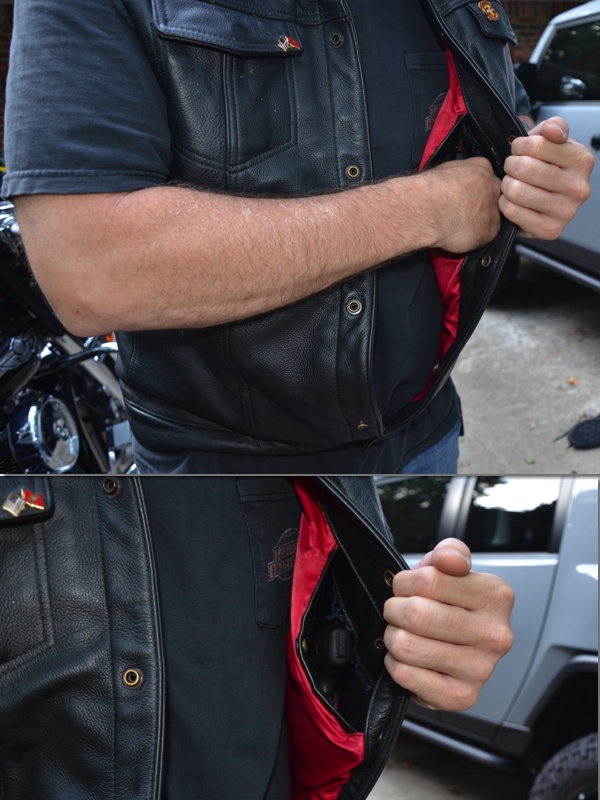In the first image, a man is depicted wearing a black short-sleeve t-shirt under a sleeveless leather vest with blue jeans. His left hand is reaching into an inner pocket of his vest, which is lined with red fabric. The second, close-up image reveals that this inner pocket is designed to conceal a gun; the butt end of the firearm is visibly nestled inside. The vest appears to be made of black leather and might have some pins attached, potentially with controversial symbols. In the background of the first image, a white truck and the outline of a black tire are visible on the right, while the left side hints at the presence of a motorcycle.